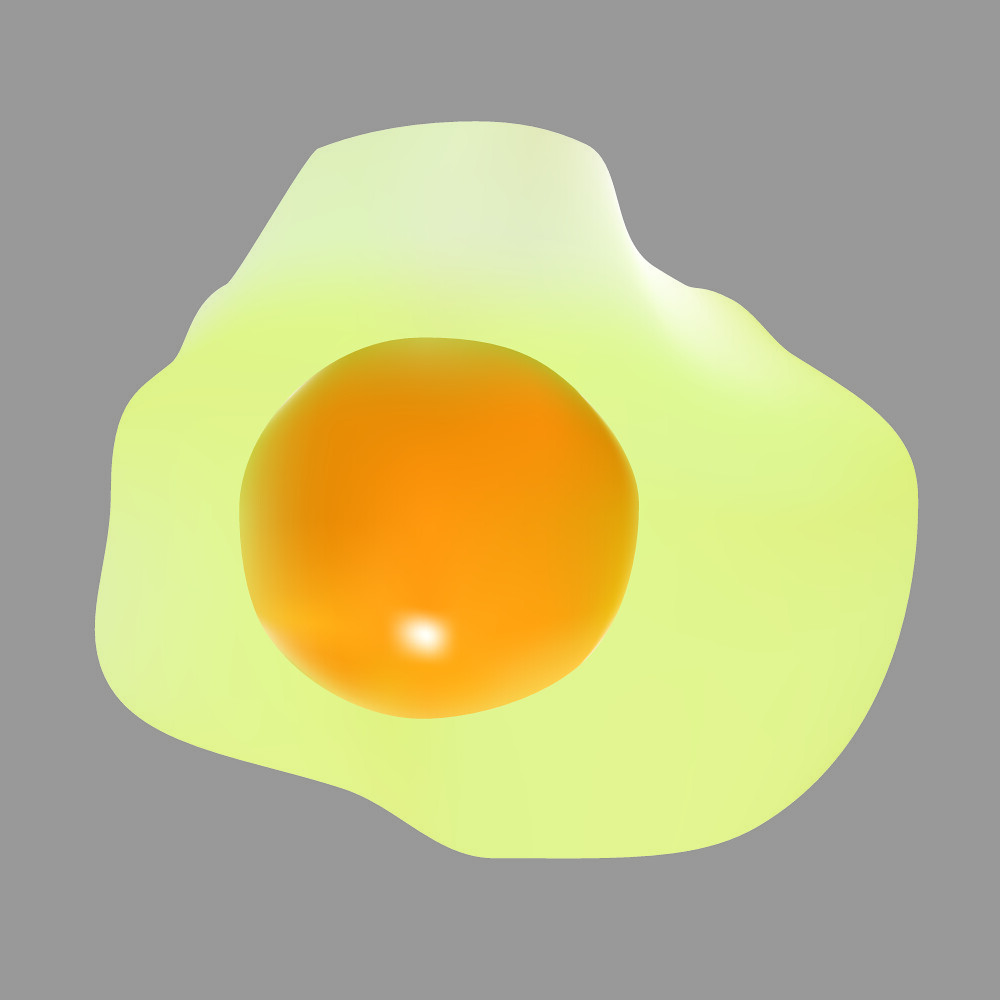This image digitally depicts a cracked-open egg with its contents spread out. At the center is a circular, dark yellow yolk, which appears slightly three-dimensional with a noticeable bulge and a light reflection at its bottom. Surrounding the yolk is an irregularly shaped albumen, primarily light yellow in color with some areas appearing plain white. The background of the image is light brown or grey, emphasizing its computer-generated nature. The digital style of the depiction gives the egg a two-dimensional appearance, particularly in the way the whites and yolk are rendered.